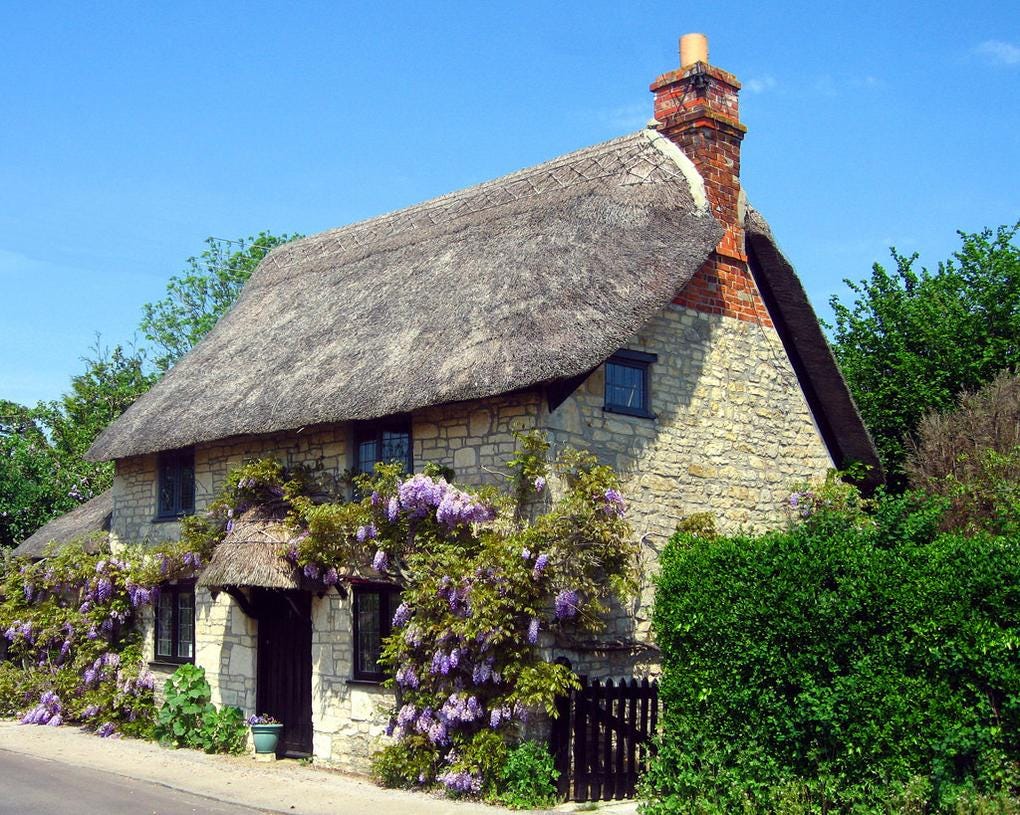This color photograph, presented in landscape orientation, is a picturesque depiction of a fairy tale-like two-family thatched roof cottage set in the serene countryside under a clear blue sky dotted with a few clouds. The cottage, angled with its corner facing the viewer, has a sloping roof of gray shingle-like thatch materials resembling a rug and includes a red brick fireplace chimney capped with brass.

The facade of the house is constructed from cream-colored stones with gray joints, creating a quaint, timeless aesthetic. The front wall elevation faces the bottom left side of the image, where an entrance door with a small covered roof of brown-gray thatch material is centrally located. The doorway is flanked by shrubs and adorned by cascading purple wisteria vines and lilac bushes that add a burst of color and charm. An aqua-colored stone planter filled with greenery is situated near the door, contributing to the lush surroundings.

Above the doorway, an arched wooden thatched roof further enhances the cottage's enchanting appearance. On the lower level, two windows with black wooden frames and two additional windows directly above provide ample light to the interior. The chimneys, windows, and doors are harmoniously integrated into the stone surface, blending beautifully with the overall rustic aesthetics of the house.

Surrounding the cottage are well-maintained green shrubs and a fence made of foliage, which includes a slightly open black picket gate that invites you into the front yard. A paved gray road and a white sidewalk lead up to the house, adding to the peaceful countryside scene. The lush greenery, colorful flowers, and meticulous details make this image a stunning representation of photographic realism.